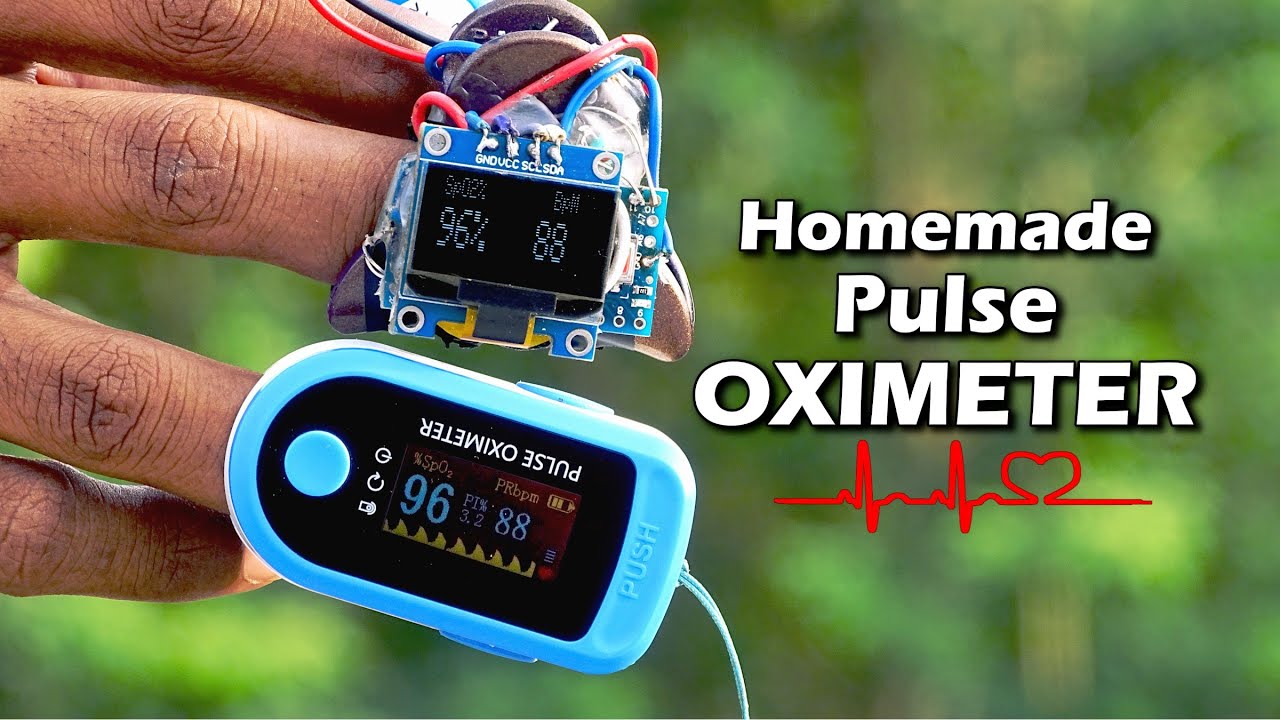The color photograph prominently showcases a detailed comparison between a homemade pulse oximeter and a commercial one on a hand. The hand extends from the left side of the image, revealing only the fingers, which are positioned against a blurred green background that hints at plants and an outdoor setting. The hand has a dark brown complexion, and it is adorned with devices on two fingers.

On the top finger, there is a homemade pulse oximeter featuring red and blue wires trailing off the screen. The device displays "SP02% 96" and "BPM 88" on a black panel. Below it, clipped to another finger, is a commercial pulse oximeter that has the same readings: "96% oxygen level" and "88 pressure," with "pulse oximeter" inscribed on its turquoise blue casing. The device's screen is black and it has a turquoise button on the side.

Hovering on the right side of the image, in large white text, the caption reads, "homemade pulse oximeter," accompanied by a red EKG-like diagram that transitions into a heart shape before flattening out. The image appears to be a screenshot or thumbnail for a video, emphasizing the hands-on comparison of these devices.